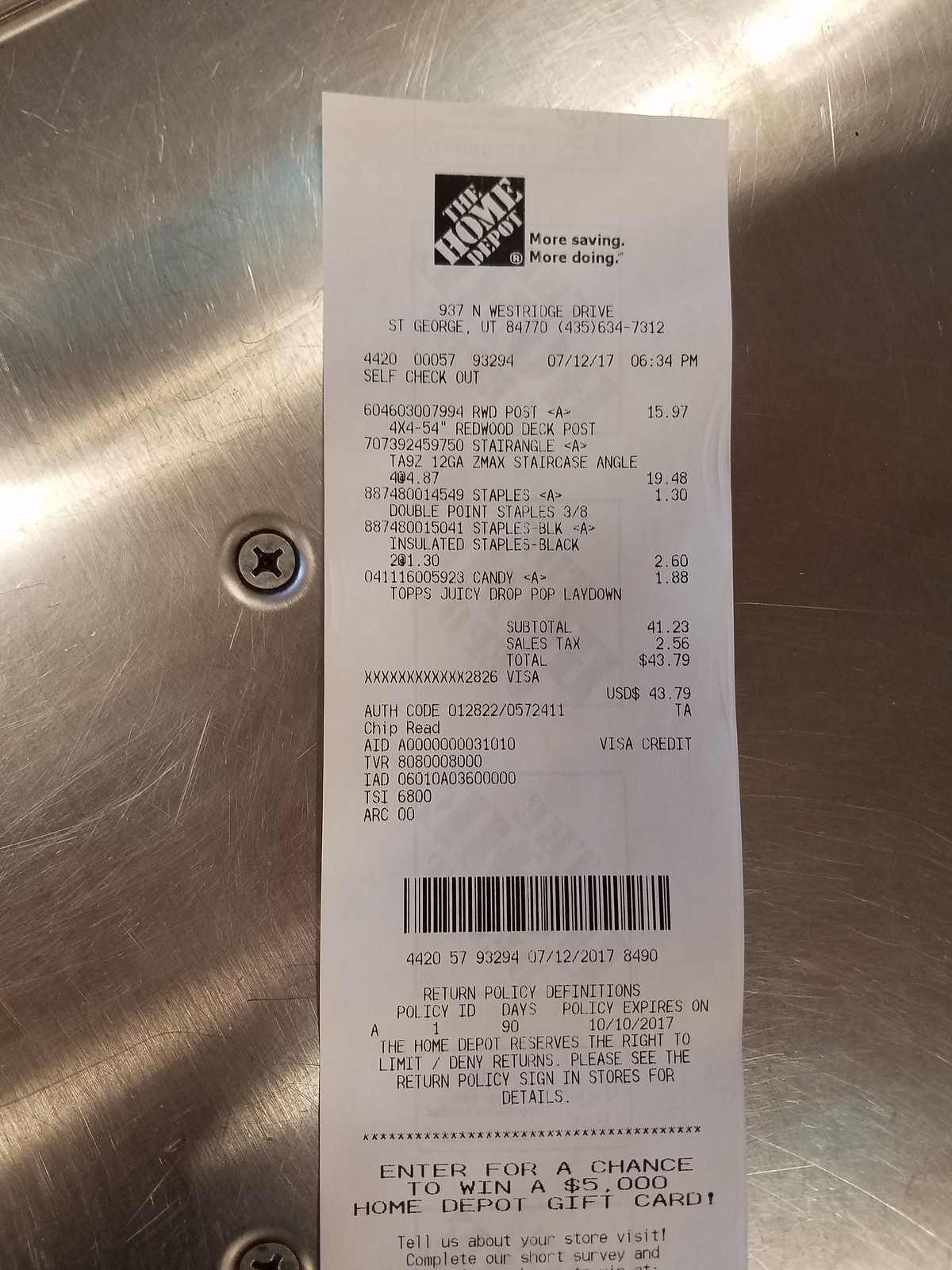The image shows a Home Depot receipt placed on a metallic table surface, which is visibly scratched and has two screws on it. The receipt features the Home Depot logo—a black square with white diagonal lettering—followed by the slogan "More Saving. More Doing." written next to it on the right side. Below, the store's address is listed as 937 Westridge Drive, St. George, Utah, 84770, with the contact number 435-634-7312.

Highlighted on the receipt are several transaction details:
- A transaction ID: 4420-000-5793-294
- Date and time of purchase: July 12, 2017, at 6:34 PM
- Another reference number: 604-603-000-7994

The items purchased are as follows:
1. Redwood Deck Post (4x4-54") with product code 70739-2459-750, priced at $15.97.
2. Staircase Angles (12GA ZMAX), quantity of 4, at $4.87 each, summing to $19.48.
3. Double Point Staples (3/8"), one pack at $1.30.
4. Insulated Black Staples, two packs at $1.30 each, totaling $2.60.
5. A Juicy Drop Pop Laydown candy, listed for $1.88.
 
The subtotal amounts to $41.23, with a sales tax of $2.56, bringing the total to $43.79. The purchase was made using a Visa credit card.

The bottom of the receipt outlines Home Depot's return policy, indicating the return period, with policy definitions and expiration date mentioned as October 10, 2017. Additionally, it mentions a chance to win a $5,000 Home Depot gift card by participating in a short survey about the visit.